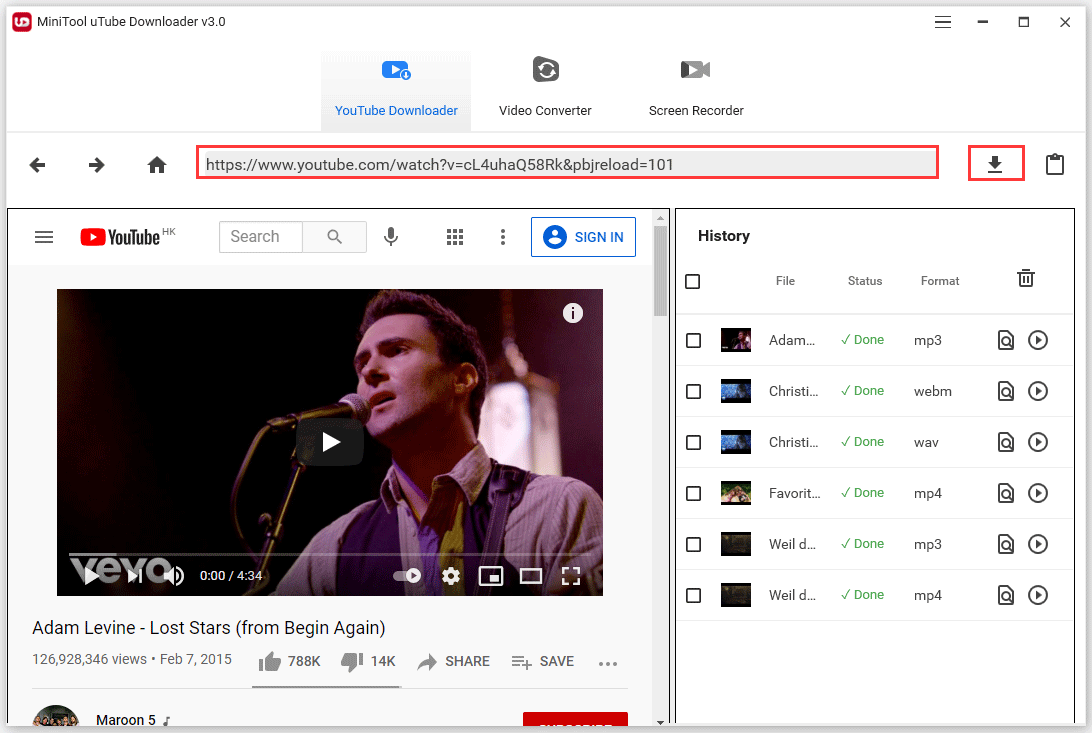In this screenshot, a user interface of the MiniTool YouTube Downloader version 3.0 is displayed, showcasing its streamlined layout for downloading YouTube videos. The top section of the interface prominently features the MiniTool YouTube Downloader 3.0 branding. Below this, several primary tabs can be observed, including "YouTube Downloader" (currently selected), "Video Converter," and "Screen Recorder."

The main area is divided into two sections. On the left, there is a URL input field containing a paused video URL, indicating the user has interacted with it recently to check its availability. Adjacent to this field, a prominent "Download" button is positioned.

Beneath the URL field, a thumbnail and details of the YouTube video "Lost Stars" by Adam Levine from the movie "Begin Again" are visible. The video is illustrated as having gained significant traction with 788,000 likes and 14,000 dislikes, emphasizing its popularity. 

On the right side of the interface, there is a "History" section where the user can manage previously downloaded videos. The layout is noted for its user-friendly design, clearly segmenting the input, video preview, and download history areas—ensuring a clean and organized experience for the user.